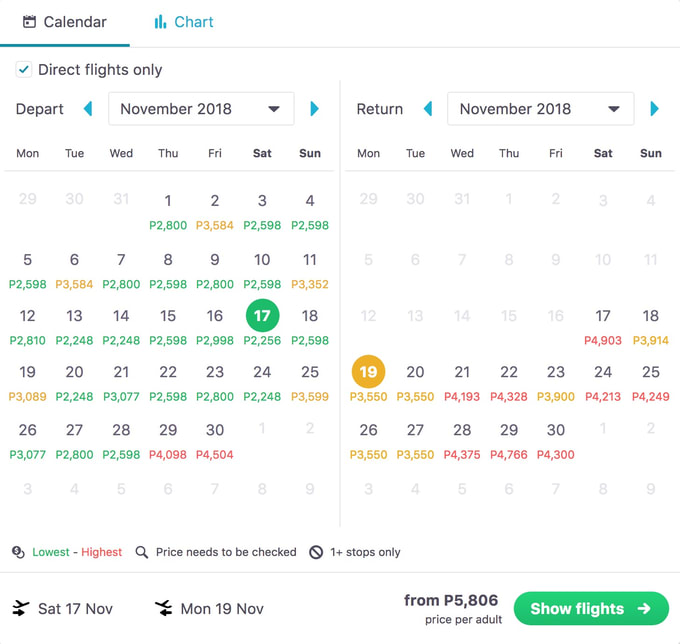The image is a screenshot of a flight search page, captured in a slightly vertically rectangular frame. At the top left corner, against a white background, two options labeled "Calendar" and "Chart" are displayed side by side. The "Calendar" option is currently selected, indicated by a teal horizontal line beneath it. Below these options, there's an option labeled "Direct Flights Only" with a checked box beside it.

The primary content features two calendars side by side, both for November 2018. The calendar on the left is marked as "Depart" and has November 17th circled in green, indicating the selected departure date. The calendar on the right is labeled "Return" and has November 19th circled in orange, denoting the chosen return date. Each date on the calendars displays various alphanumeric entries, such as P2, P2800, and P3584, which likely represent different flight options, prices, or categories, though their specific meanings are unclear.

At the bottom right of the image, there is a prominent green button labeled "Show Flights," inviting the user to proceed with viewing available flight options.